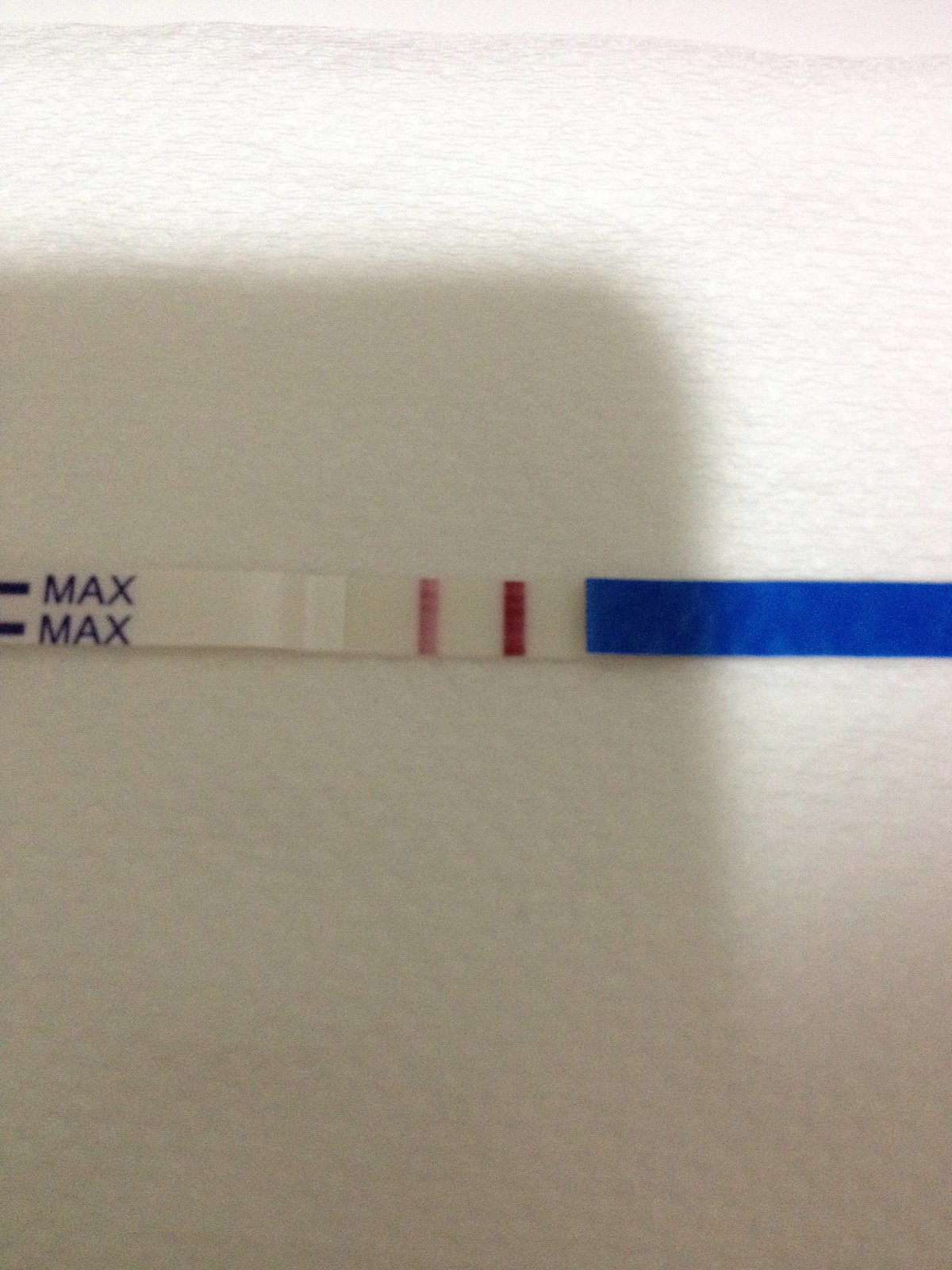This image features a photograph in portrait orientation, showcasing a test strip laid out on a white background, which appears to be either a cloth or a paper towel. The lighting casts a shadow over the bottom part of the image, creating a tall rectangular shape, reminiscent of a cell phone shadow, that bisects the scene.

The test strip, oriented horizontally from left to right, is marked by specific elements and colors. On the left side of the strip, it displays two blue lines—one at the top and one at the bottom—accompanied by the capitalized blue word "MAX". 

Moving towards the center of the strip, there is a light red vertical line followed by a darker red vertical line against a white background. These colored lines seem to be the primary indicators of the test results. The strip transitions to a solid blue color on the right third, completing its journey across the page.

The strip's design indicates its purpose for diagnostic or result-reading usage, with the white and shiny areas highlighting around the "MAX" labels, contrasted by the non-shiny center where the test results are visible.